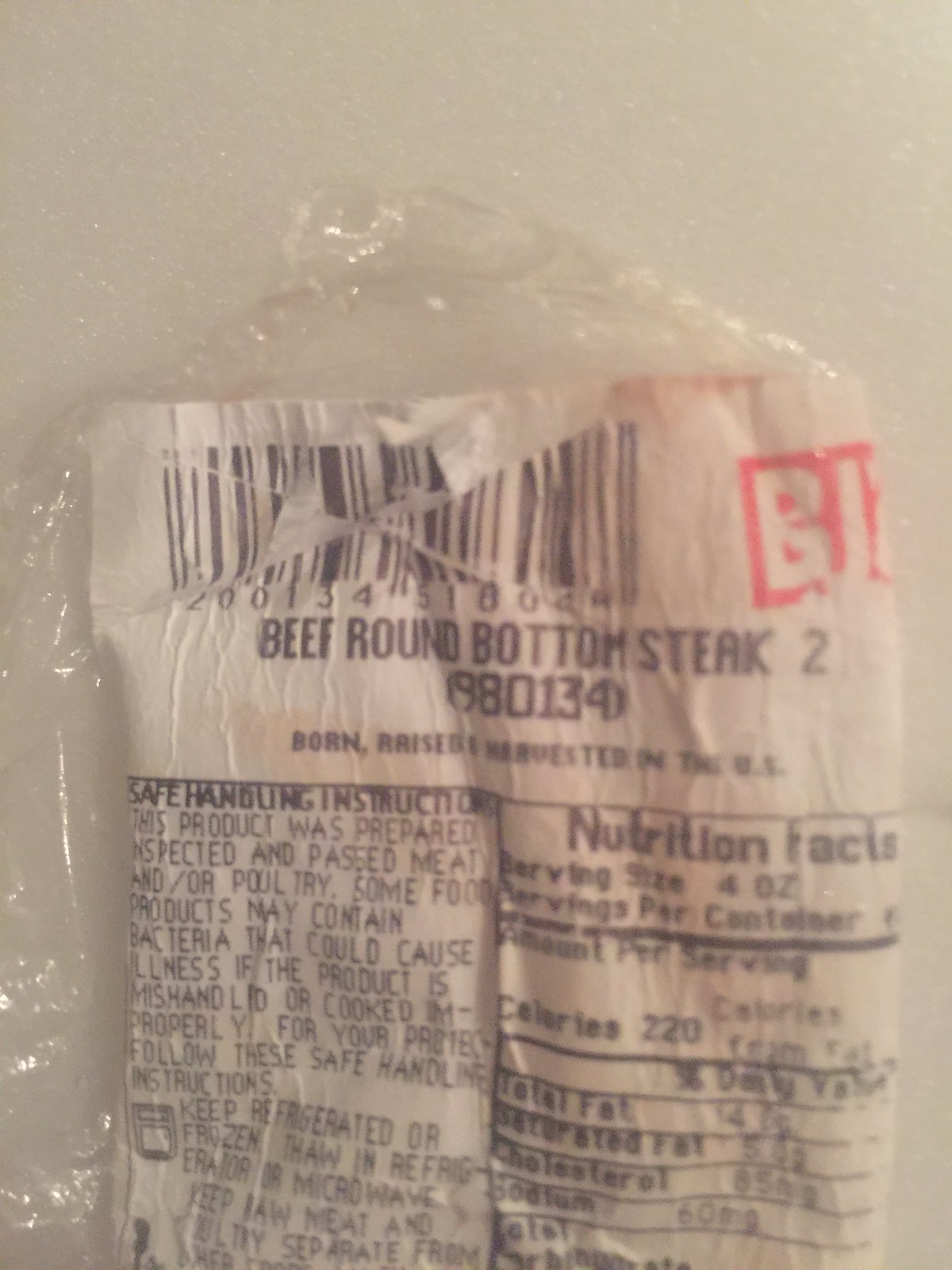The photograph captures a torn piece of saran wrap with an attached white label set against a plain white background. The label, originally from a meat package, features detailed information in black font. It reads: "Beef Round Bottom Steak," followed by a product code, "2, 980134," and the assurance that the meat was "born, raised, and harvested in the United States." Below this text, a black line divides the label. On the right side of the label, there are nutritional facts, while the left side contains cooking instructions for the meat. This image seems to document the front label of a meat package that has been torn off for emphasis or record-keeping.